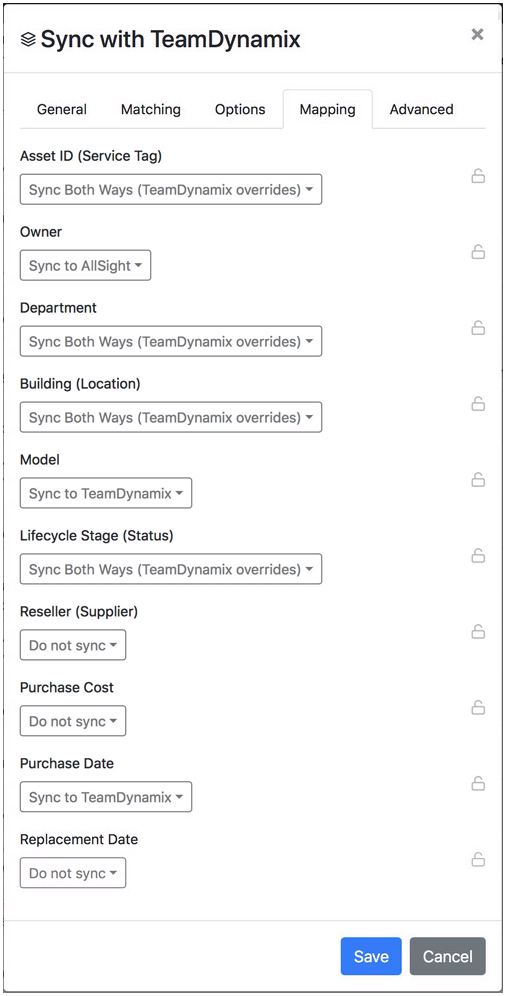The screenshot depicts a management application interface viewed on a cell phone in portrait orientation, with a height approximately twice its width. The visual outline includes a thick border at both the top and bottom, as well as a thinner gray border on the right side. 

At the very top, there is a slender green separator line beneath which lies a white background section featuring black text that reads "Sync with Team Dynamics." Accompanying this text is an icon depicting a stack of papers with an overlaying 'X' symbol.

Below this section, there are clickable options labeled: General, Matching, Options, Mapping, and Advanced. Out of these, ‘Mapping’ is highlighted with a box, indicating it is currently selected.

In the main content area, several titles with corresponding drop-down boxes are presented. The titles and their default drop-down selections are as follows:
- **Asset ID** 
- **Service Tag** with "Sync Both Ways"
- **Owner** with "Sync to All Sites"
- **Department** with "Sync Both Ways"
- **Building Location** with "Sync Both Ways"
- **Model** with "Sync to Team Dynamics"
- **Lifecycle Stage** with "Sync Both Ways"
- **Reseller** with "Do Not Sync"
- **Supplier** with "Do Not Sync"
- **Purchase Cost** with "Do Not Sync"
- **Purchase Date** with "Sync to Team Dynamics"
- **Replacement Date** with "Do Not Sync"

These entries are followed by a thin gray dividing line. At the bottom, there are two interactive buttons: a blue box with the text "Save" in white, and a gray box labeled "Cancel." Each item in the list is accompanied by a lock icon situated to its right, suggesting some form of access control or restriction.

Overall, this interface seems dedicated to managing synchronization settings for various asset details within the application, particularly aligning with "Team Dynamics."